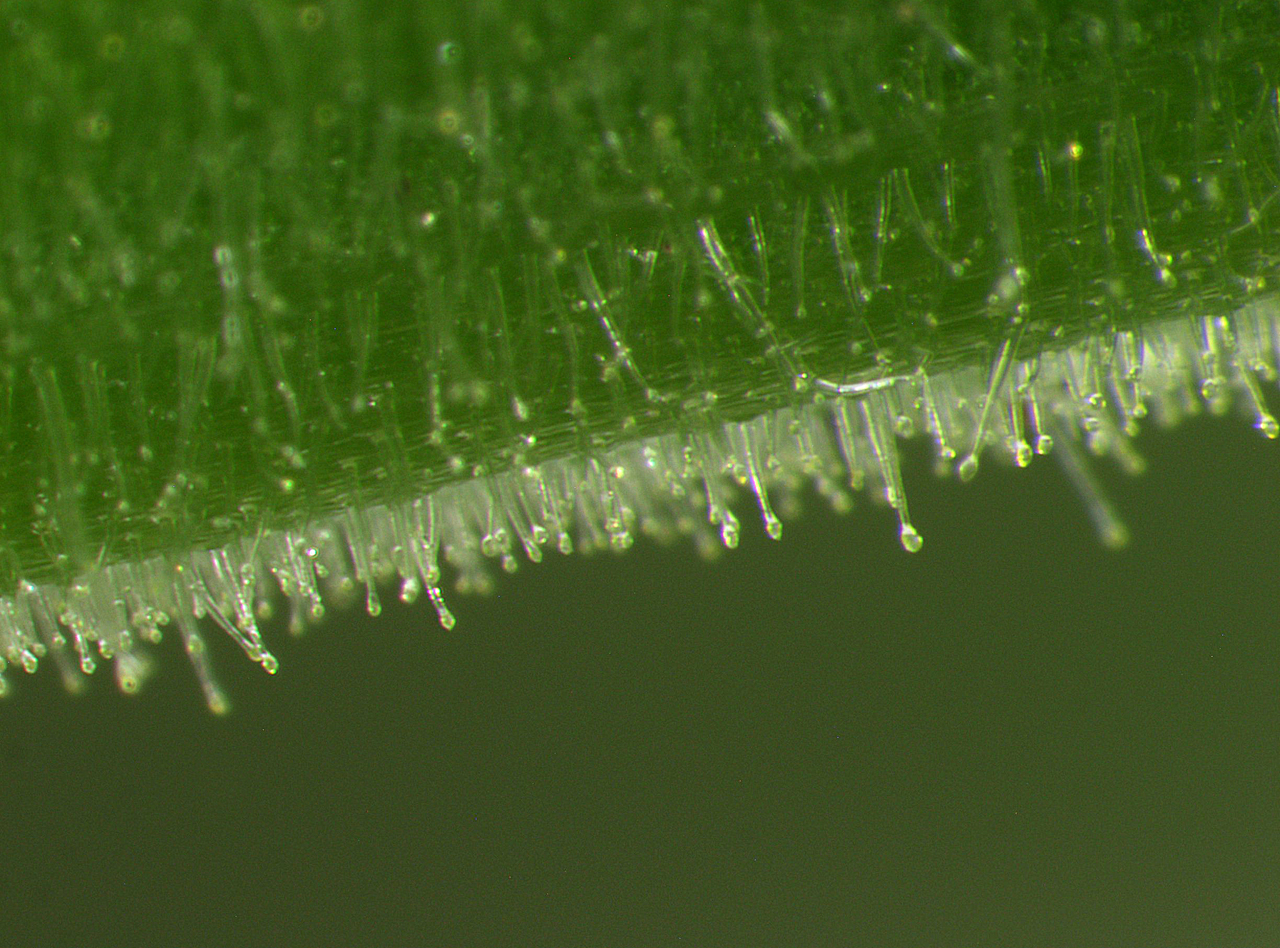The image features a striking scene of a green leaf encrusted with icicles, giving it a breathtaking, crystallized appearance. The upper portion of the image showcases the leaf, covered in a delicate layer of ice that shimmers like frost in the sunlight. Below this, a series of icicles hang down at an angle, as if the image has been rotated slightly clockwise by 20 degrees. The bottoms of the icicles and the area immediately below them transition into a dark, murky green reminiscent of algae-filled lake water, creating a contrasting backdrop. The entire scene exudes a mesmerizing, almost surreal quality, blending elements of nature and frozen beauty in a captivating, diagonal composition.